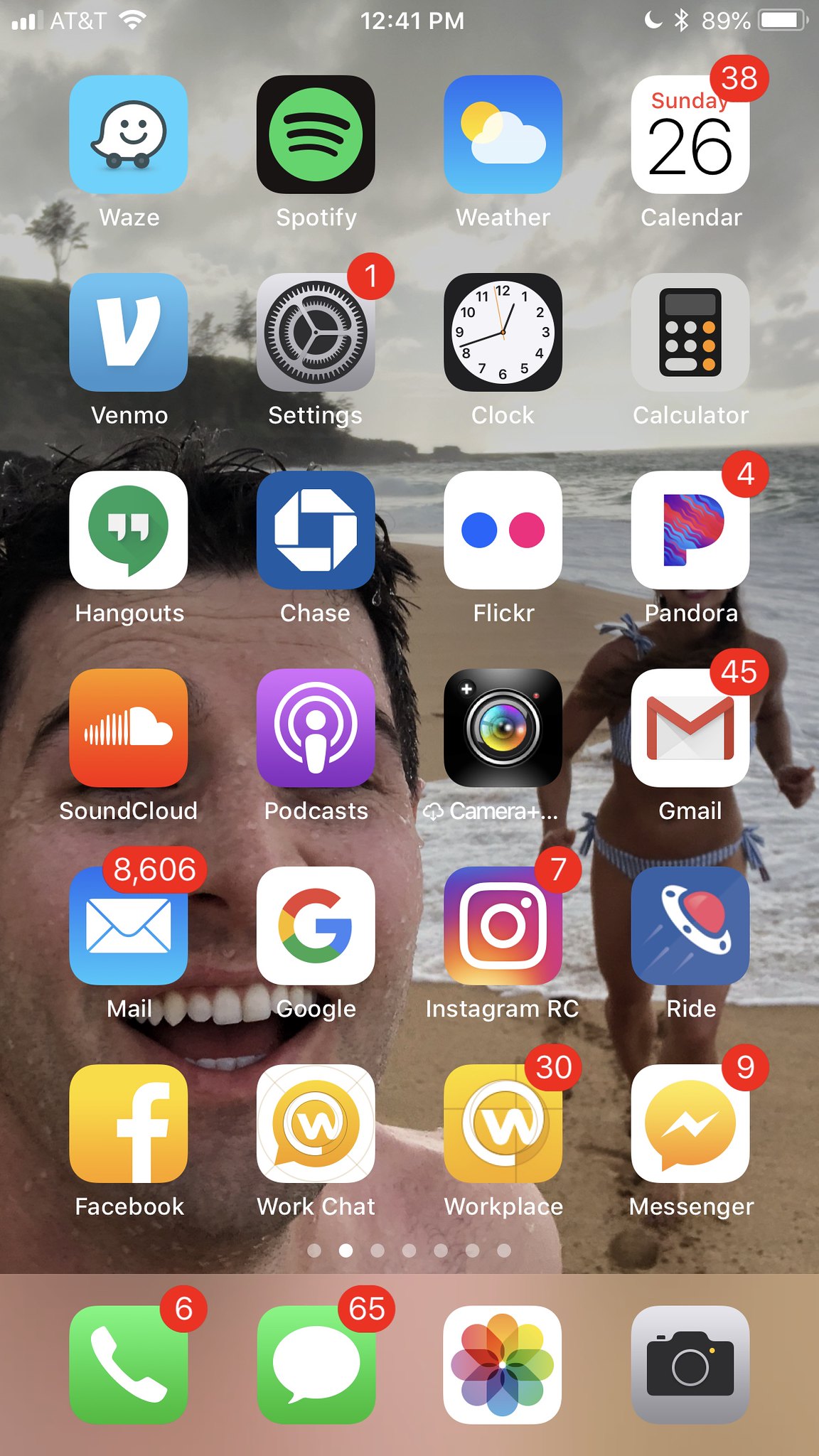A screenshot of a smartphone home screen, with an indistinguishable Android or iOS operating system, displays a grid layout of various applications. The wallpaper is a selfie taken at the beach, featuring a person in the foreground. Behind them, a girl in a blue swimsuit is visible, set against an overcast sky. Mountains and trees rise in the background to the left side of the image, just above the man's head.

The apps are organized in rows of four from left to right, starting with:
1. **Waze**, **Spotify**, **Weather**, **Calendar** (with 38 notifications on Calendar).
2. **Venmo**, **Settings** (with 1 notification), **Clock**, **Calculator**.
3. **Hangouts**, **Chase**, **Flickr**, **Pandora** (with 4 notifications).
4. **SoundCloud**, **Podcast**, **Camera**, **Gmail** (with 45 notifications).
5. **Mail** (with a staggering 8,606 notifications), **Google**, **Instagram** (with 7 notifications), **Ride RC**.
6. **Facebook**, **WorkChat**, **Workplace** (with 30 notifications), and **Messenger** (with 9 notifications).

Below these, there are four more unlabeled but commonly identified apps: **Phone** (with 6 notifications), **Messages** (with 65 notifications), **Photos**, and **Camera**.

This detailed layout highlights an organized yet busy digital life with numerous pending notifications across various communication and social platforms.